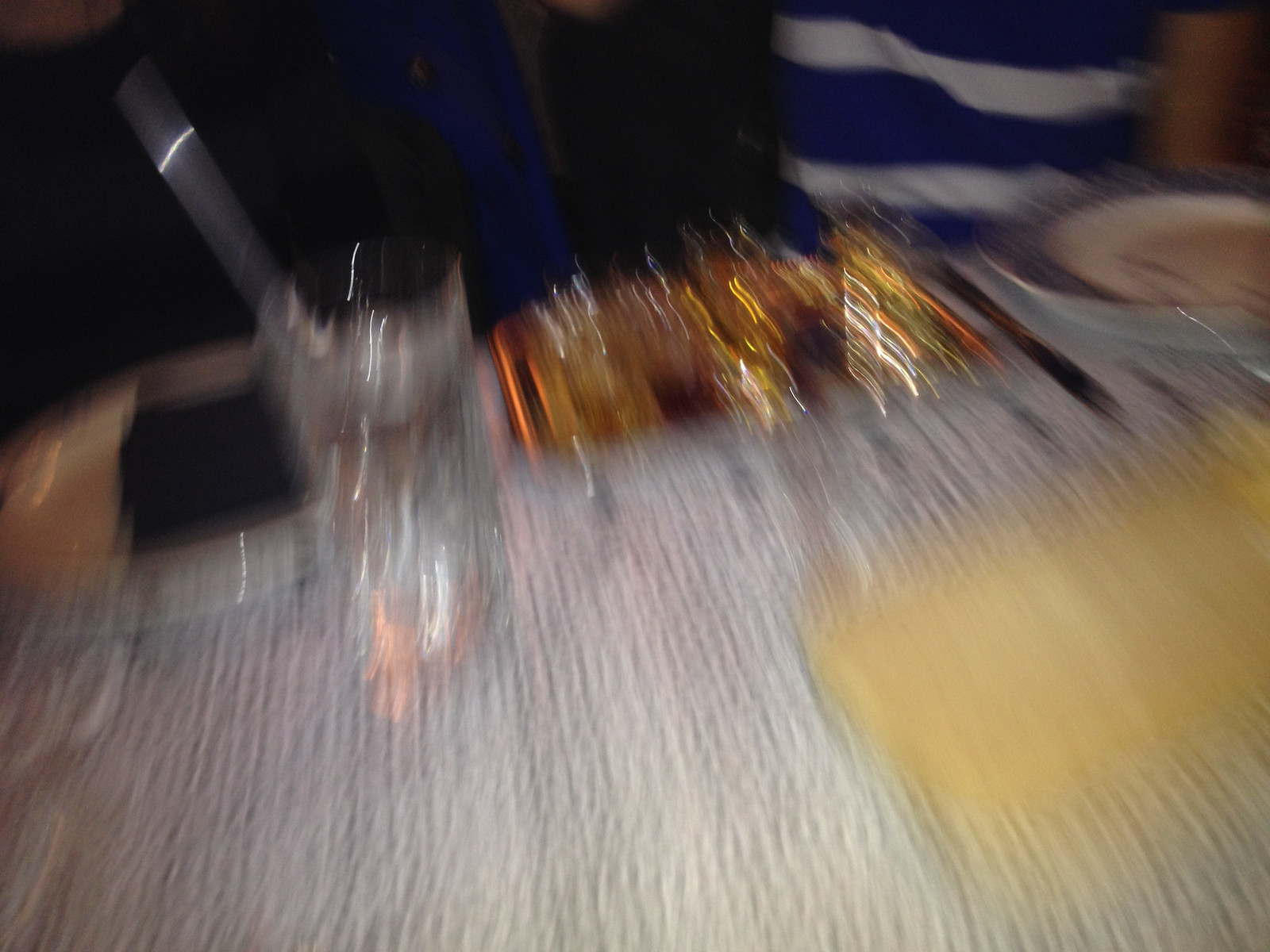This highly blurred photograph depicts a table setting that is challenging to discern with certainty due to the extreme lack of clarity. The table is covered with a white tablecloth and features a yellow placemat. On the opposite side of the table, a plate is visible, accompanied by some cutlery. Two figures can be vaguely identified: one wearing a blue and white striped shirt, and another clad in a blue shirt, seated next to each other. In front of the person in the blue shirt, there is what appears to be a glass. Positioned between the two individuals on the table is an obscure, shiny, golden, and bronze object that is very glittery and streaky, defying precise identification. Overall, elements like a possible check or wallet, and various reflections contribute to the scene's complexity. Elements within the setting, including a potential dessert-like item on a glass plate and various reflective surfaces, add to the ambient visual confusion.